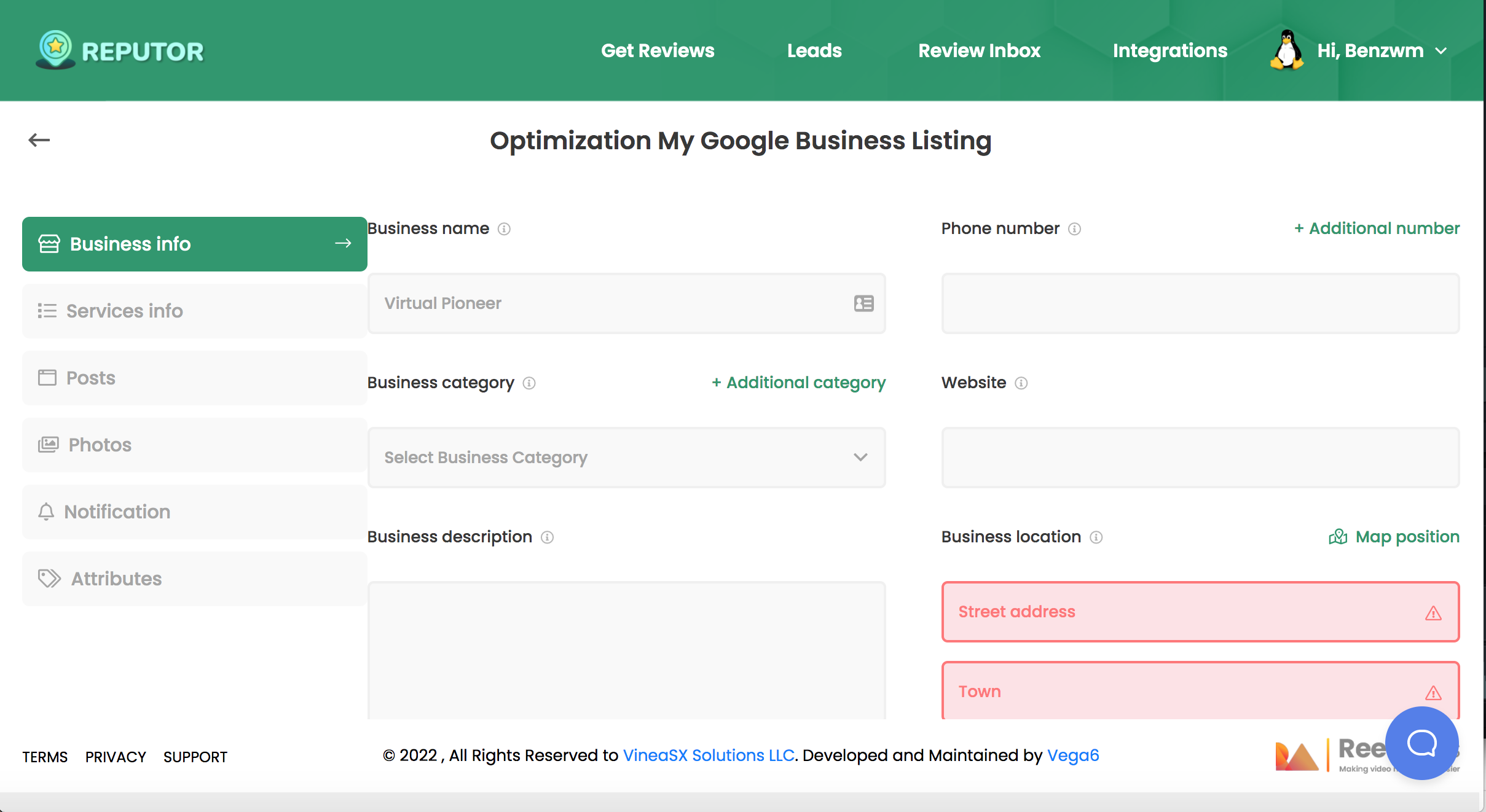**Descriptive Caption:**

The image is a screenshot of the Reputor website's interface, showcasing a variety of functional tabs and sections geared towards business optimization. At the top of the page, several navigation tabs are visible: Get Reviews, Leads, Review Inbox, and Integrations. To the right of these tabs, a whimsical graphic of a sitting penguin is present, alongside a welcome message that reads "Hi Men's Wim," likely addressing the user.

The central portion of the page focuses on "Optimization" of the user's Google Business Listing. Along the left side, a vertical list of tabs is displayed. The currently active tab, "Business Info," is highlighted in a green box, while other tabs include Services Info, Posts, Photos, Notification, and Attributes.

Within the main area of the "Business Info" tab, several input fields are laid out for updating business details. The sections include:

- **Business Name:** An input field currently containing the placeholder text "Virtual Pioneer" in gray.
- **Phone Number:** A dedicated field for entering the business contact number.
- **Business Category:** An input field for specifying the category of the business.
- **Website:** A field for entering the business's website URL.
- **Business Description:** An area for providing a brief description of the business.

Additionally, there are sections for entering "Business Location" details, including Street Address and Town. Both of these fields are highlighted in red, accompanied by an error symbol indicating that the necessary information is missing.

The bottom of the page features links to the website's "Privacy" and "Support" terms, providing users with additional resources and information.